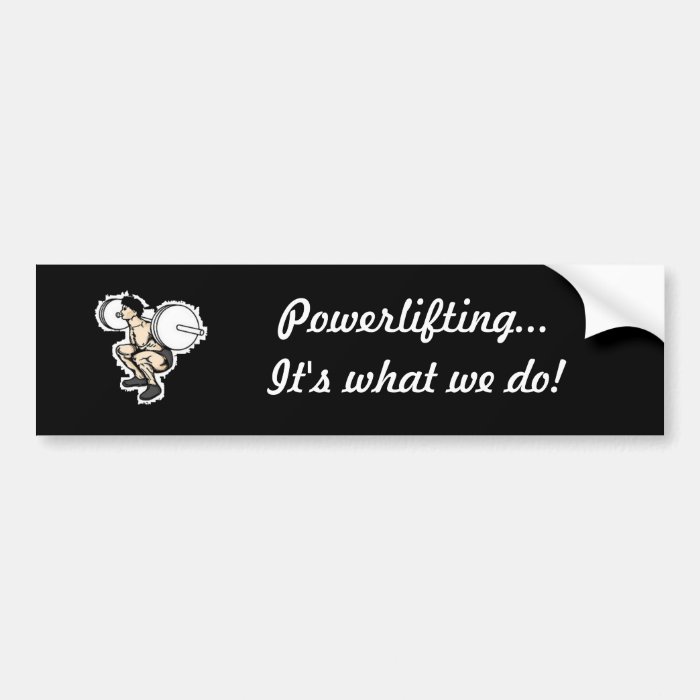The image features a white rectangle with its length longer than its width. In the center of the rectangle, there's a black banner. The banner has its top right corner folded forward, revealing a white surface underneath. On the left side of the banner, a cartoon-style logo depicts a man squatting and holding up a barbell with two circular weights. To the right of the logo, the text "Powerlifting..." is written in white, followed by a second line that reads "is what we do!" The black banner, contrasted against the light gray background of the overall rectangle, directs the viewer's attention to the central message and imagery.